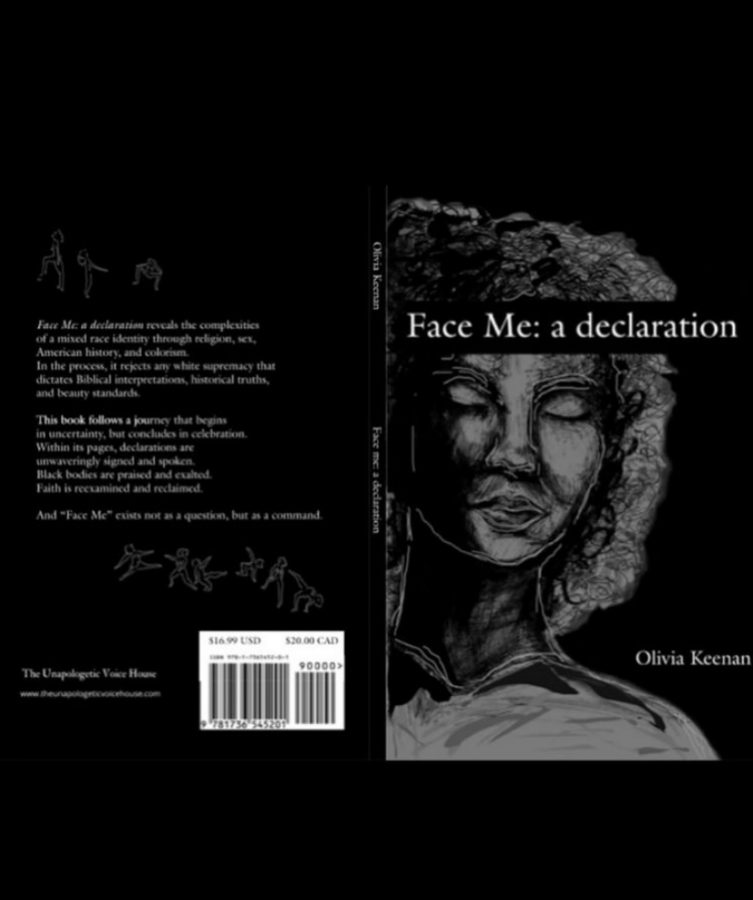The image depicts a photo scan of both the front and back covers of a book set against a completely black background. The book appears to be laid flat with the front cover on the right side and the back cover on the left. The front cover features a pencil sketch of an older African-American woman with curly hair falling to her neck. Written across her forehead in large white text is the book's title, "Face Me: a declaration," with the subtitle in lower case. The author's name, Olivia Keenan, is positioned in the bottom right, nestled in the space created by her neck and shoulders.

On the back cover, there are small black and white figurine illustrations at the top, followed by a couple of paragraphs summarizing the book's content, which discusses the complexities of mixed-race identity through various themes like religion, sex, American history, and colorism. At the bottom, there is a barcode along with the book's pricing: $16.99 USD and $20 CAD.